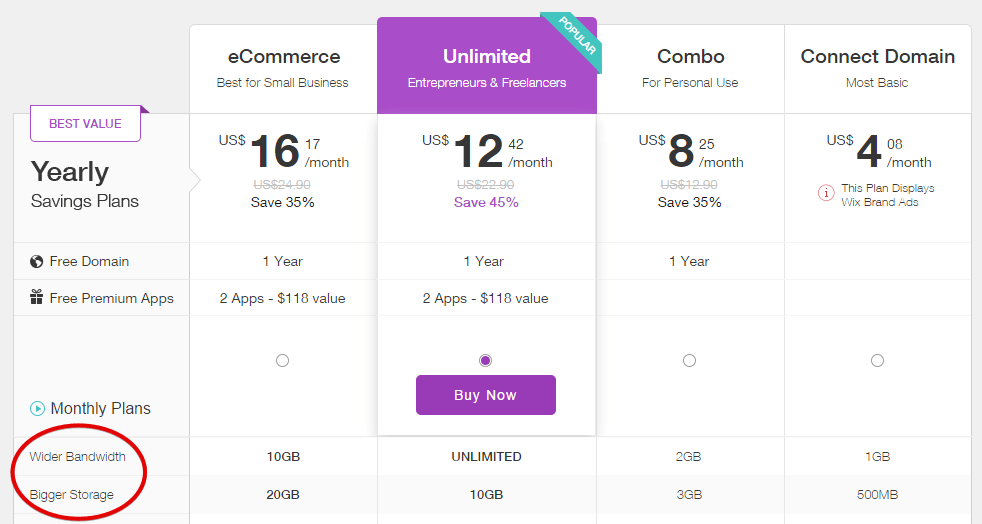**Detailed Caption:**

The chart presents various subscription plans for businesses, highlighting their features and pricing structures. On the left side, there's a "Best Value" section in purple, indicating the yearly savings associated with each plan. 

The primary categories include:
- **E-commerce (Best for Small Business)**: Priced at $16.17 per month (originally $24), offering a 35% savings. This plan includes 10 GB of bandwidth and 20 GB of storage.
- **Unlimited (Most Popular)**: At a discounted rate of $12.42 per month, it gives entrepreneurs and freelancers unlimited bandwidth and 10 GB of storage. This option is highlighted with a green bar and has a purple outline, denoting its popularity.
- **Combo (For Personal Use)**: Available for $8.25 per month, providing 2 GB of bandwidth and 3 GB of storage.
- **Connect Domain (Most Basic)**: The simplest option at $4.08 per month, offering 1 GB of bandwidth and 500 MB of storage.

Each of these plans runs for a duration of one year, except for the Connect Domain plan. Additionally, the E-commerce and Unlimited plans include two apps with a combined value of $118. Other features across the plans include options like free domain, free premium apps, wider bandwidth, and increased storage capacities, with certain benefits circled in red for emphasis.